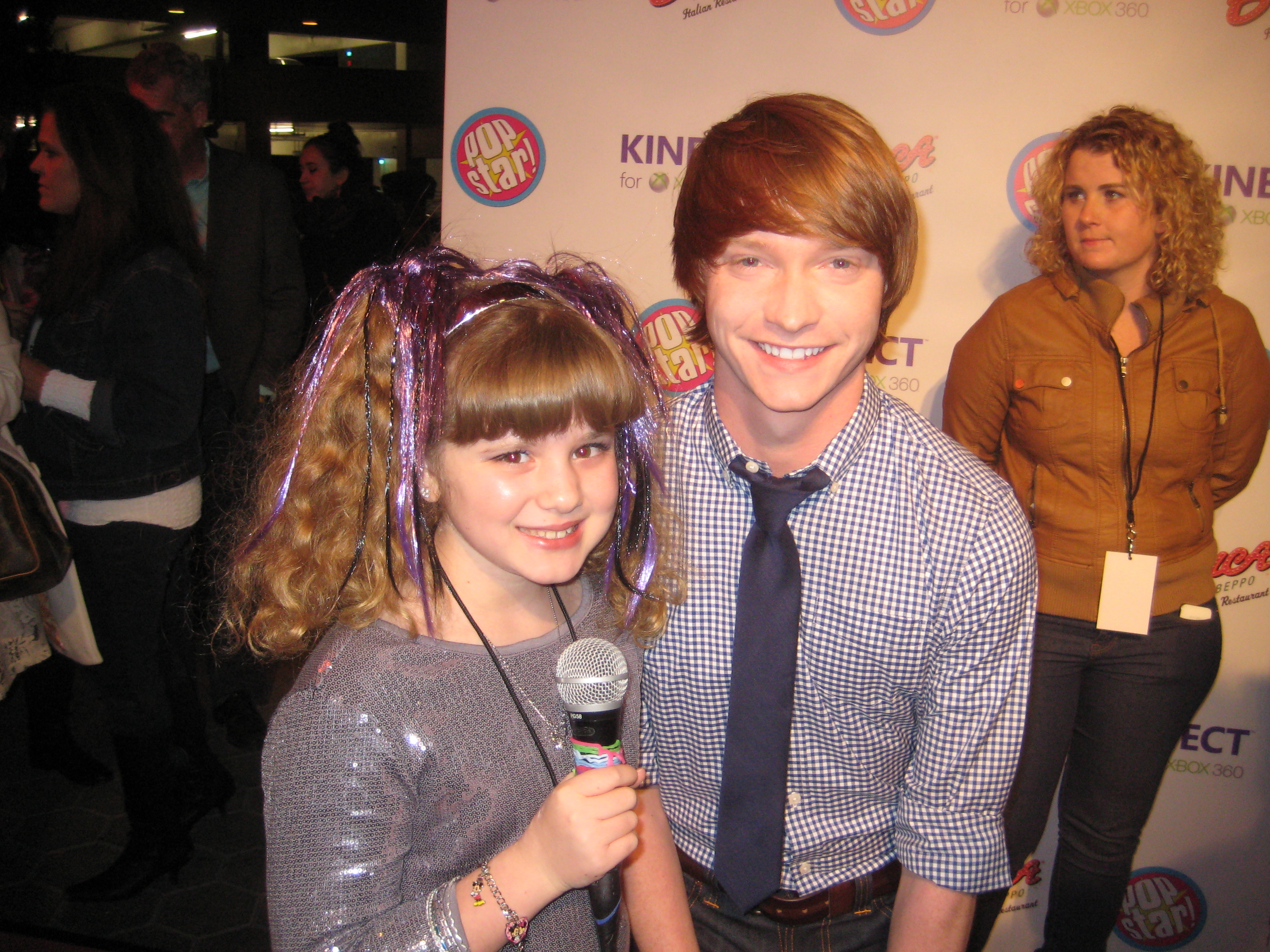The image depicts a lively event, presumably a gathering for young pop stars or actors. At the center is a young girl, possibly a child actress, with purple ribbons in her curly brown hair. She is holding a microphone and wearing a sparkly gray top. Beside her is a slightly older boy with short dirty blonde hair. He smiles broadly while dressed in a distinctive blue tie with a houndstooth-patterned shirt, sleeves rolled up. In the background stands a woman with curly blonde hair, dressed in a bright brown shirt, a long jacket, and blue jeans. She wears a lanyard with a white tag around her neck. Behind them, there is a white display that prominently features the word "pop star" and another word beginning with "K" in purple. Multiple people are scattered around, observing the scene, adding to the bustling atmosphere of the gathering.